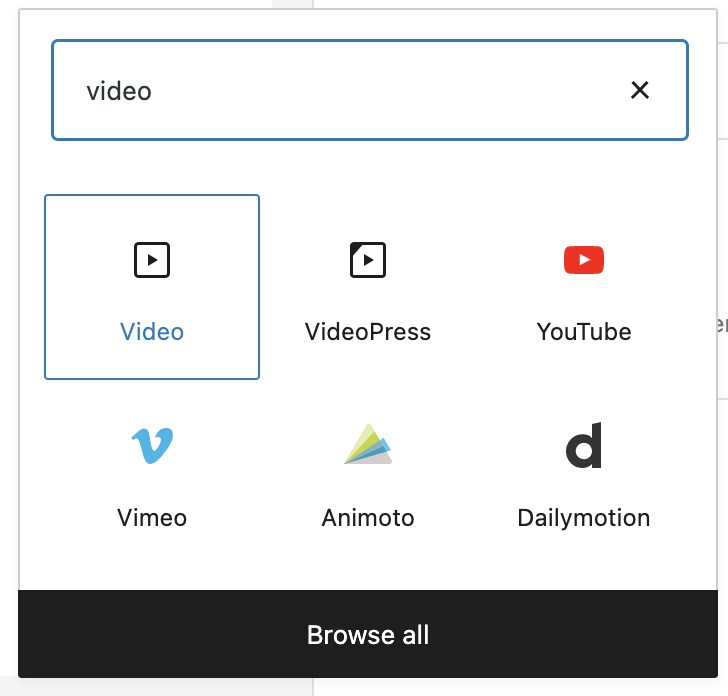The image displays an app interface with the title "Vito" prominently featured at the top. The background at the top of the page is white, and within this section, the text "Vito" is written in black inside a blue-outlined rectangle. Below this titled section, there are six distinct buttons arranged vertically.

1. The first button is highlighted and labeled "Vito" in blue, enclosed within a blue square outline.
2. The second button reads "Vito Press," accompanied by an icon depicting Vito Play.
3. The third button is labeled "YouTube," featuring the recognizable red YouTube logo with a play button at its center.
4. The fourth button, positioned on the bottom left, is labeled "Vimeo" and includes a blue 'V' icon.
5. The fifth button is named "Animoto" and is illustrated with a colorful triangle icon in shades of green, light green, blue, and grey.
6. The sixth and final button is titled "Dailymotion," accompanied by a black 'D' icon.

At the bottom of the page, a button labeled "Browse All" appears. This button features white text on a black background, contrasting with the overall white background of the top section of the app page.